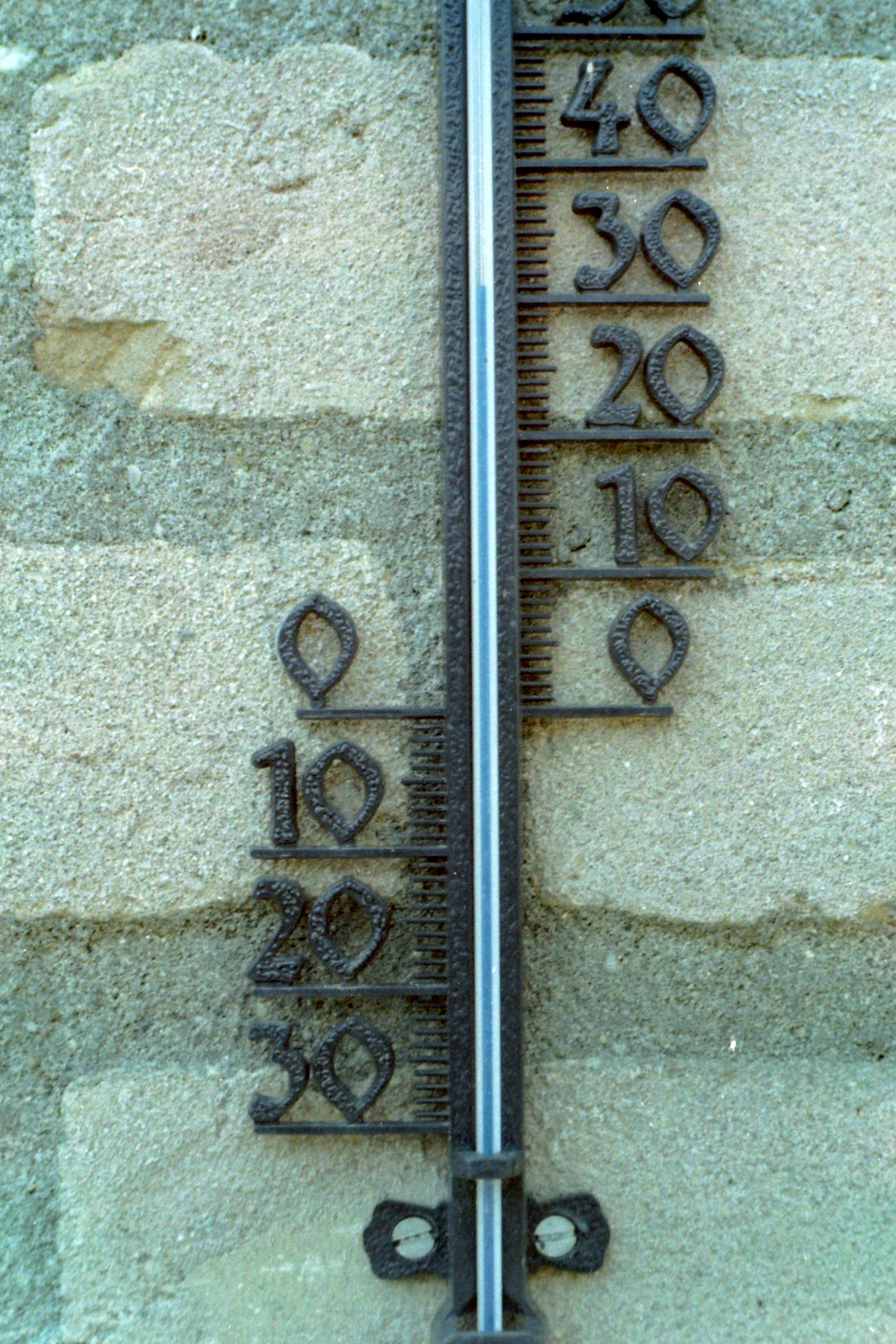The image features a predominantly gray-colored brick wall that serves as the background. Centrally, there is a prominent vertical arrangement consisting of three lines: a thick white line flanked by thinner black lines on either side. Approximately 80% up the white line, a vertical blue line intersects it, extending from the bottom to about 80% of the way up, leaving the top 20% of the white line unobstructed.

To the right of the central lines, starting from the top, a sequence of numbers descends vertically. The topmost number, likely 50, is partially obscured, followed by clearly visible numbers 40, 30, 20, 10, and 0, each accompanied by a shorter black horizontal line aligned with the middle of the digits. Additionally, there are nine smaller black tick marks to the left of each number, creating a sense of precision and measurement.

On the left side, a matching series of numbers begins at 0 and descends as 0, 10, 20, and 30. These numbers are also connected by shorter black horizontal lines, stretching only as far as the digits themselves, taking up approximately 20-30% of the horizontal space on that side.

At the bottom of the image, directly beneath the central vertical line assembly, two screws are visible—one on each side of the central black line—embedded in black plastic fittings, adding a functional, industrial element to the overall composition.